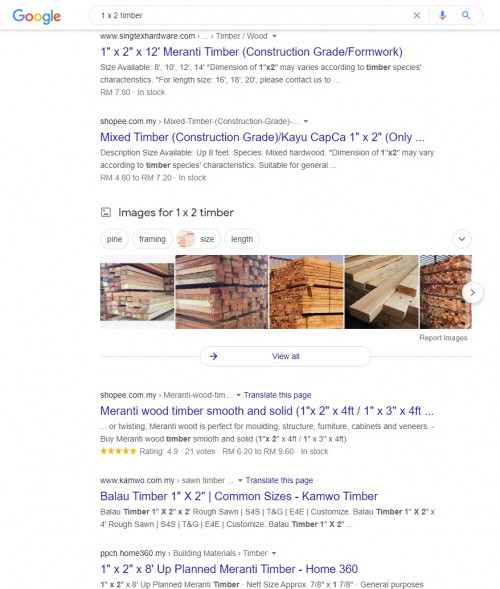A screenshot of Google search results for "1 by 2 timber" is displayed. The search query is visible in the search bar. The top search result is "1 by 2 by 12 Maranti timber, construction grade/formwork." Following this, the second result reads "Mixed timber construction grade, Caillou Capca, 1 by 2." The third result offers "Maranti wood timber, smooth and solid, 1 by 2 by 4 feet / 1 by 3 by 4 feet." The subsequent listing is for "Baillieu timber, 1 by 2, common sizes, Commonwealth timber." The final search result highlights "1 by 2 by 8 Upland Maranti timber."